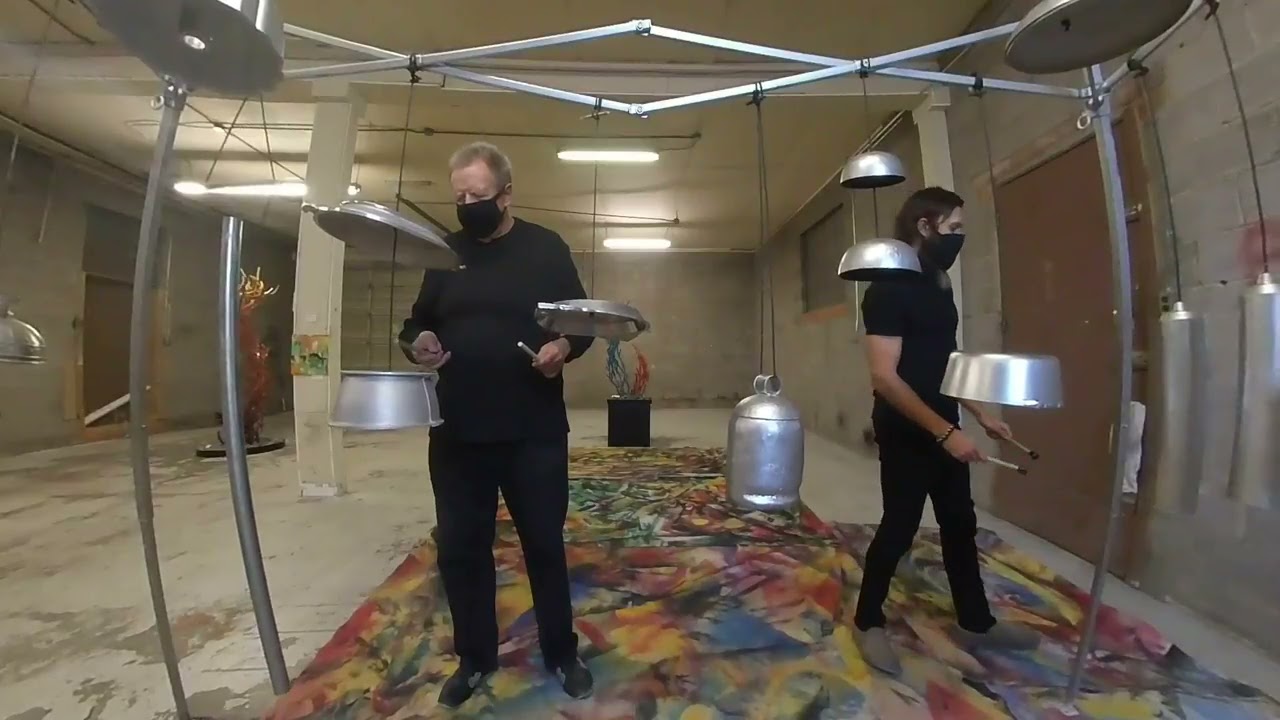In this image, two men are standing in an expansive, beige room with a slightly distorted, fisheye effect. Both men are dressed entirely in black, including masks. The older man on the left has short blonde hair, a long-sleeved black shirt, black pants, and black shoes with grey patches. The younger man on the right wears a half-sleeved black shirt and black pants, with grey shoes. Both are holding drumsticks and mallets, and each stands before a metal contraption that features various suspended metal items, including pots, pans, bowls, and lids, all silver in color. The contraption has poles that rise from the ground, supporting a criss-cross metal bar at the top. Beneath them is a vibrant, multi-colored, abstract rug. In the background, a simple, beige cement wall and floor are visible, along with a decorative object on a black pedestal featuring blue and red branch-like structures. Some lights are mounted on the ceiling, highlighting the room's minimalistic decor.